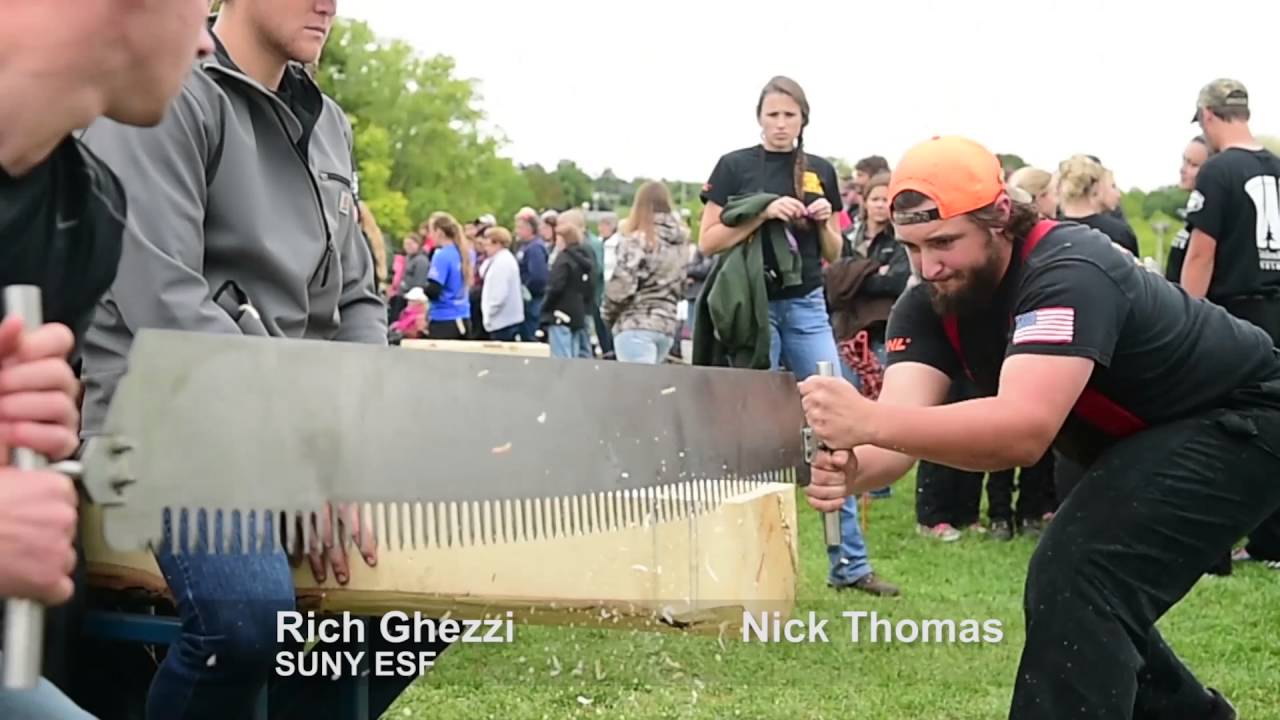In a lush green pasture surrounded by trees, a large group of people is gathered. At the center of the photograph, two men are working together with a large saw, cutting a small section from a thick, long piece of wood. The man on the right is clearly visible; he has brown hair and a brown beard, wears a black t-shirt with an American flag on his left sleeve, and the letters "NL" partially visible on his right sleeve. His orange baseball cap is worn backward, and a caption identifies him as Nick Thomas. The second man is partially cropped out of the photograph, with only his hands and part of his head visible, suggesting he might be wearing a dark jacket. His caption reads Rich Gezzi, SUNY ESF. Nearby, a third man in a gray jacket and blue jeans sits on the log, steadying it. A woman in a black shirt, carrying a green jacket and dressed in blue jeans and dark boots, watches the activity from behind. The background reveals a crowd of people extending back, some engaged in conversation while others watch the sawing demonstration. The sky above appears whitish, adding a neutral backdrop to the vibrant scene below.